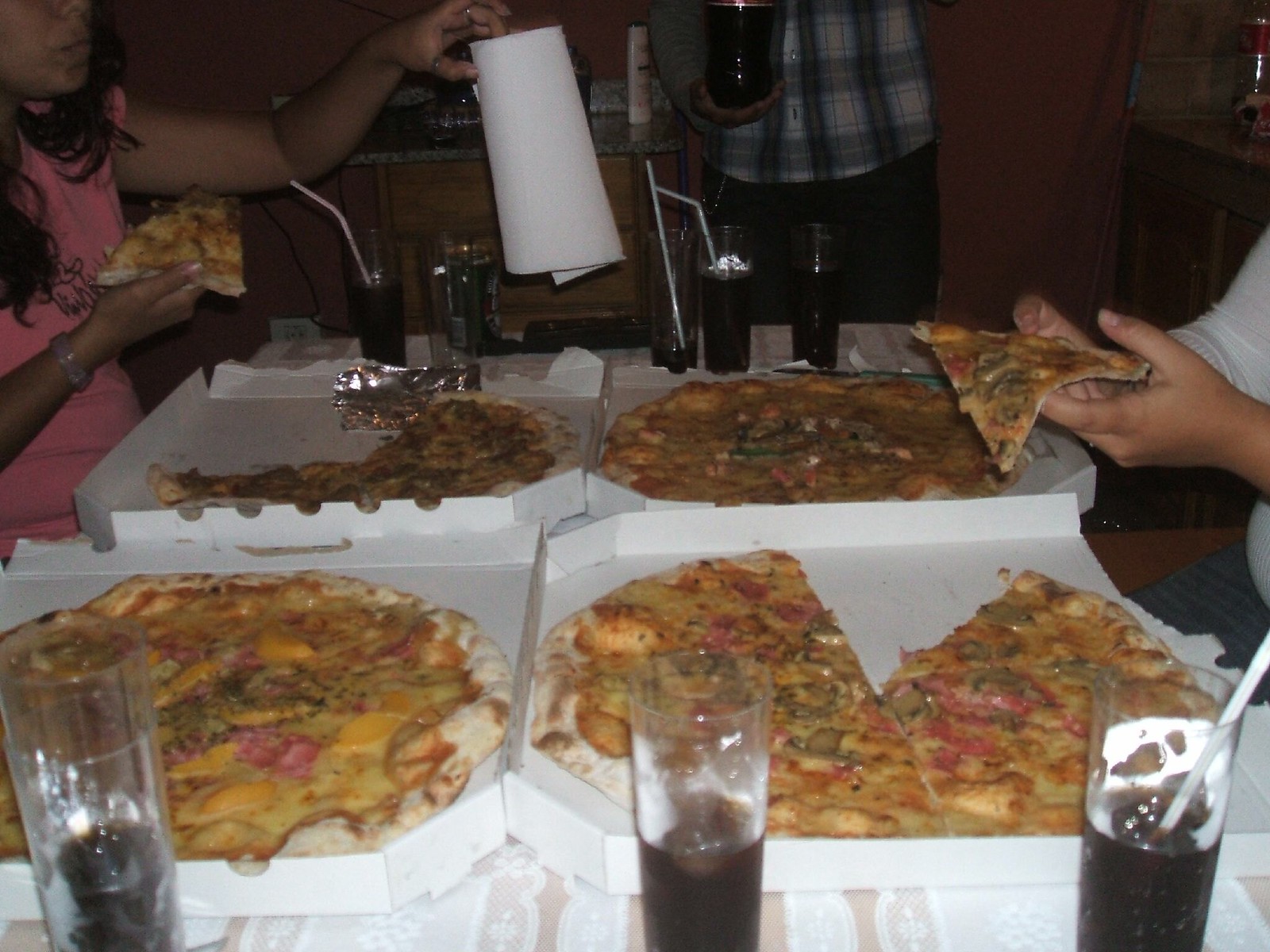This image captures a nostalgic pizza party scene reminiscent of the 70s or early 80s, characterized by its vintage photo quality. At the forefront of the image sits a table laden with four pizzas, each notably detailed with light brown crusts, vibrant yellow cheese, and assorted toppings including brown mushrooms and red tomatoes. 

From the top left of the image, a person with dark hair in a coral-colored shirt holds a slice of pizza in their right hand, with a bracelet adorning their wrist, while their left hand clutches a roll of paper towels. To their immediate right, another individual in a grey checkered shirt is seen holding a bottle of soda. At the far right, another person is depicted, wearing a grey top and pants, holding a slice of pizza.

On the table beneath these individuals, four open pizza boxes are arranged, some pizzas partially eaten. In the immediate foreground, three clear glasses each contain a dark beverage, likely soda; the glass on the far right includes a white straw. In the background, five additional glasses are visible, three of which are also filled with the dark liquid and have straws protruding from them. The use of flash in the photography accentuates the front of the frame, adding a dimensional contrast to the image.